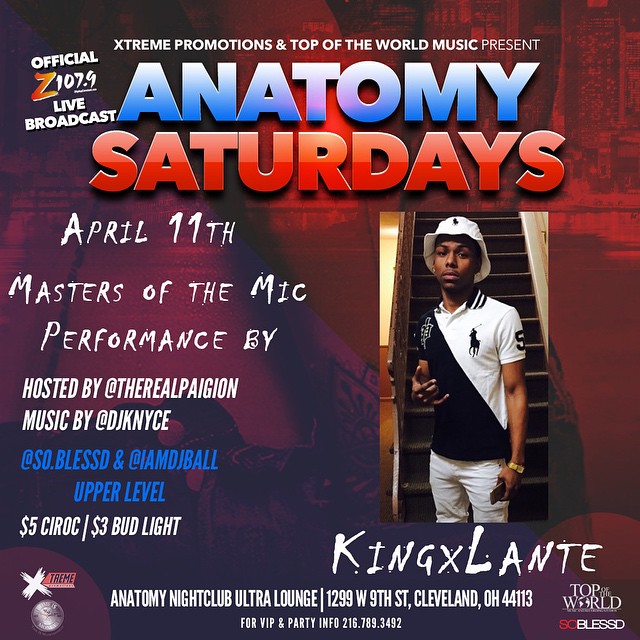This vibrant advertisement promotes a live broadcast on Z107.9 for "Anatomy Saturdays" on April 11th, titled "Masters of the Mic." Sponsored by Extreme Promotions and Top of the World Music, the event features performances hosted at The Real Pagan with music by DJ Knice, So Blessed, and J Ball Upper Level. The flyer prominently showcases beer prices—$5 C-Rock and $3 Bud Light—underneath a photograph of a young black man in a white hat, white pants, and a polo shirt, identified as King X Lante. The bottom section lists the venue as Anatomy Nightclub Ultra Lounge in Cleveland, Ohio, and provides contact information for VIP and party details at 216-789-3492. The advertisement, set against a red-toned cityscape, includes logos for Extreme, Top of the World, and So Blessed on either side.